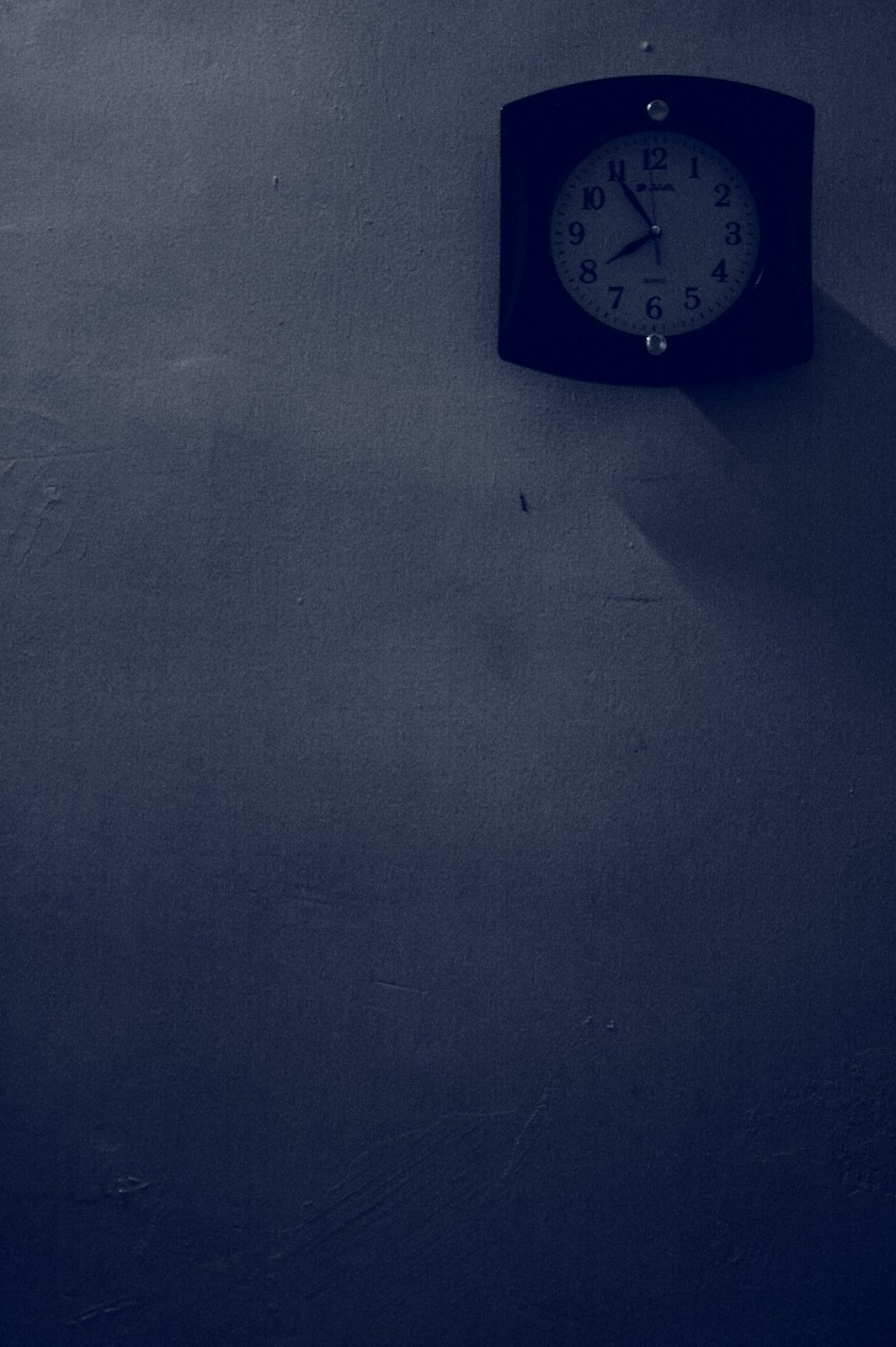The image depicts a very dark, rough-textured wall that appears to have shades of gray and black, suggesting it might be plaster and possibly old or poorly maintained. The focal point is a clock mounted high on the upper right-hand side of the wall. The clock features a distinctive design, with a white round face encased in a frame that's square-ish with rounded top and bottom edges, likely made of wood or perhaps a dark material that could also be brown. The clock's face is clearly visible with black hour and minute hands, alongside a sweeping second hand. Additionally, the clock has two round silver screws at the top and bottom, likely for mounting purposes. The time on the clock reads five to eight. The wall itself has multiple black marks and a prominent white dot located directly above the 12 o'clock position on the timepiece.